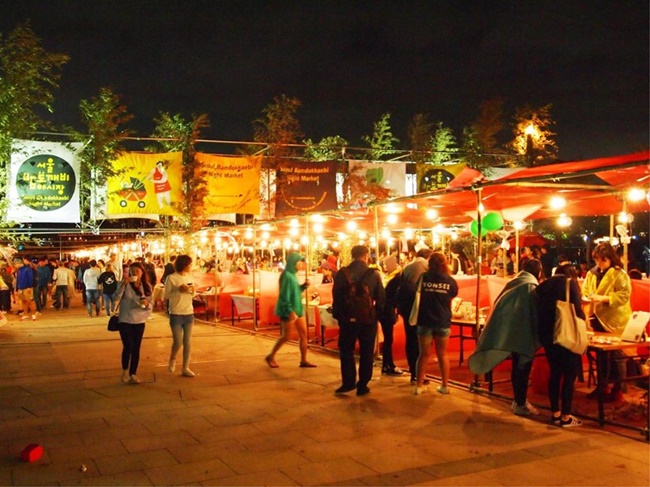The image captures a bustling nighttime outdoor festival lined with vibrant activity. The scene features numerous vendors beneath red canopy tents adorned with white and yellow lights, creating a festive glow. Casual-dressed festival-goers in hoodies, jeans, shorts, and leggings meander along a rectangular brick walkway, dotted with occasional litter. In the foreground, people line up, possibly for food or merchandise, while a woman interacts with two others near green balloons. Above the rows of booths, multi-colored banners with foreign writing are suspended from a metal frame, high enough for easy visibility. These banners, along with treetops visible in the background, contribute to the lively atmosphere. The festival extends backward, growing more crowded, with tables covered in tablecloths showcasing various goods and foods.